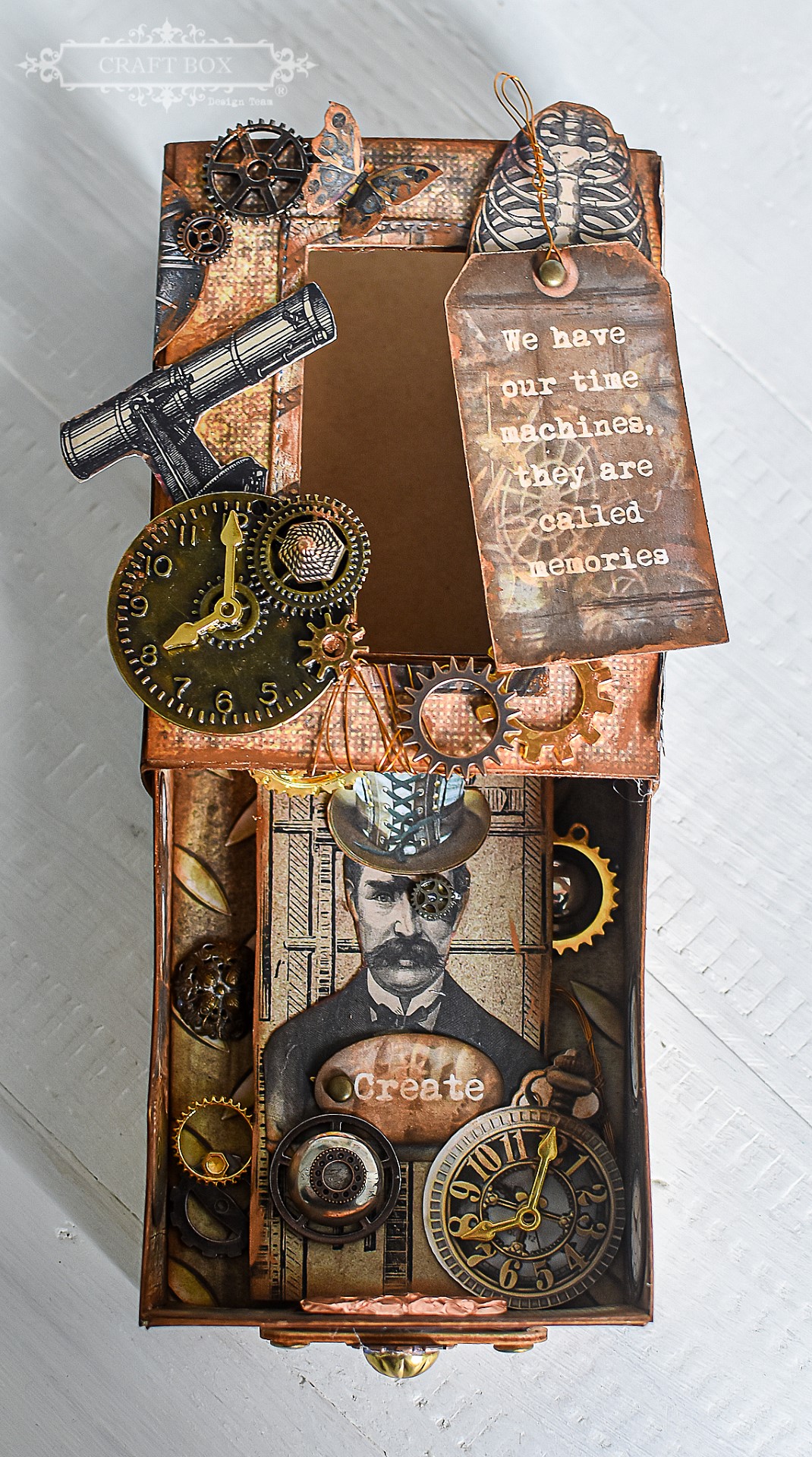This photograph captures an intricately crafted art piece rendered from a cardboard box, designed to function like a drawer that can be slid out from its exterior casing. The entire creation boasts a vintage steampunk aesthetic, meticulously adorned with various elements that ooze old-world charm and industrial allure. 

The exterior and interior surfaces of the box are embellished with an array of paper butterflies, exuding a whimsical touch. Small metal gears are strategically placed to reinforce the steampunk motif, alongside the prominent face of a clock which adds a sense of timelessness. 

A striking image of a man donning a top hat catches the eye; notably, the top hat is laced up, and a gear ingeniously replaces his monocle — a clever nod to steampunk fashion. This imaginative portrait adds a layer of narrative intrigue to the piece. 

Completing the artwork is a thoughtful paper tag affixed to the box, inscribed with the profound statement: "We have our time machines. They are called memories." This poignant message invites viewers to reflect on the intersection of time, memory, and the art itself.